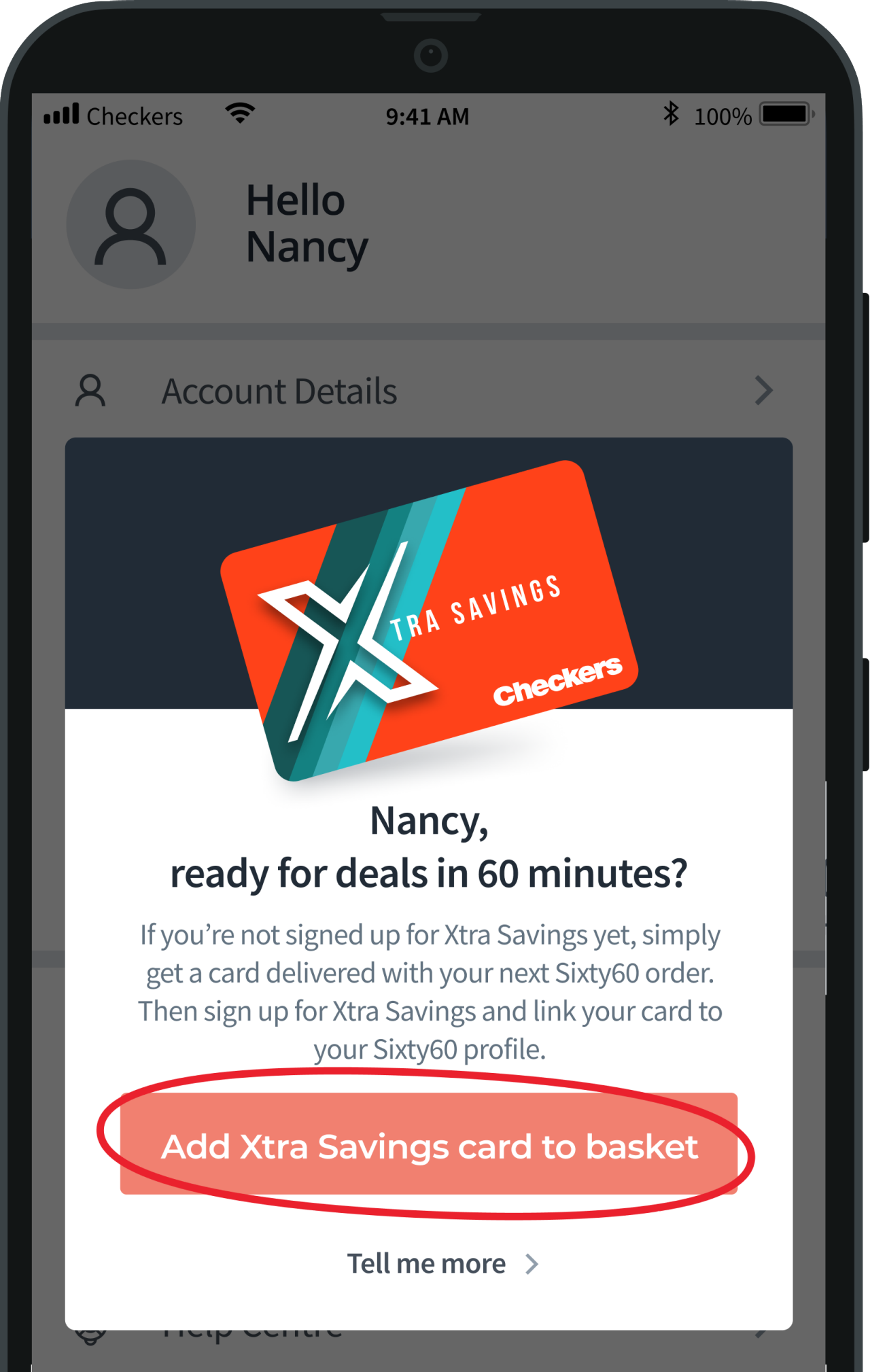Here's a detailed and cleaned-up caption for the image described:

---

A screenshot of the Checkers mobile app interface on an iPhone displays two distinct layers. The background layer features a white screen that welcomes the user with "Hello, Nancy," and includes an "Account Details" button. In the foreground, a promotional popup overlays the screen, offering Nancy deals ready in 60 minutes. The message suggests that if Nancy is not yet signed up for "EXTRA Savings" (stylized as O-E-X-T-R-A), she can simply get a card delivered with her next order of 60 units. The popup invites her to "Level Up" her savings by signing up and provides a call-to-action button for this purpose. Additionally, there's a "Tell Me More" button. The app appears to be related to Checkers, possibly a retailer providing discounts through a savings card. Notably, the promotional popup covers the entire screen with no visible close button, implying Nancy might need to tap outside the box to close it. The status bar at the top of the screen shows the iPhone is fully charged (100% battery), displaying the time as 9:41 AM, with full Wi-Fi and cellular signal strength. Beside Nancy's name, there is an outline of a male head silhouette, indicating a missing profile picture.

---